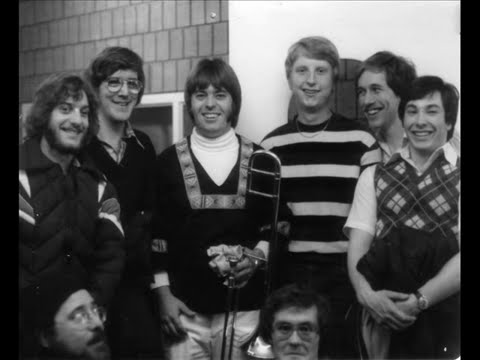This black-and-white photograph captures a group of eight young men, who appear to be in their early 20s, posing for the camera. The image likely dates back to the mid-1970s, suggested by their distinctive fashion and hairstyles. Six of the men are standing, while the other two are seated or crouched down, their heads only partially visible.

From left to right: the first man sports a full beard, curly long hair, and wears a down ski jacket reminiscent of the 70s. The next man is taller, with thick glasses and bushy hair. The central figure has long straight hair, prominent sideburns, and smiles directly at the camera, donning a white turtleneck beneath a dark V-neck sweater with a rectangular pattern. To his left stands a man holding a trombone. Three more men on the right are also smiling, with two looking directly at the camera and one gazing at the trombone holder.

The men exude a cheerful and convivial atmosphere, possibly attending a social gathering or a party, suggested by their ease and lively expressions. Their attire includes various sweaters, one notably sleeveless and argyle-patterned, and another with stripes. The backdrop features a mix of white and brick walls, possibly indicating a college setting. This snapshot vividly encapsulates a moment of camaraderie among young men in the 70s.